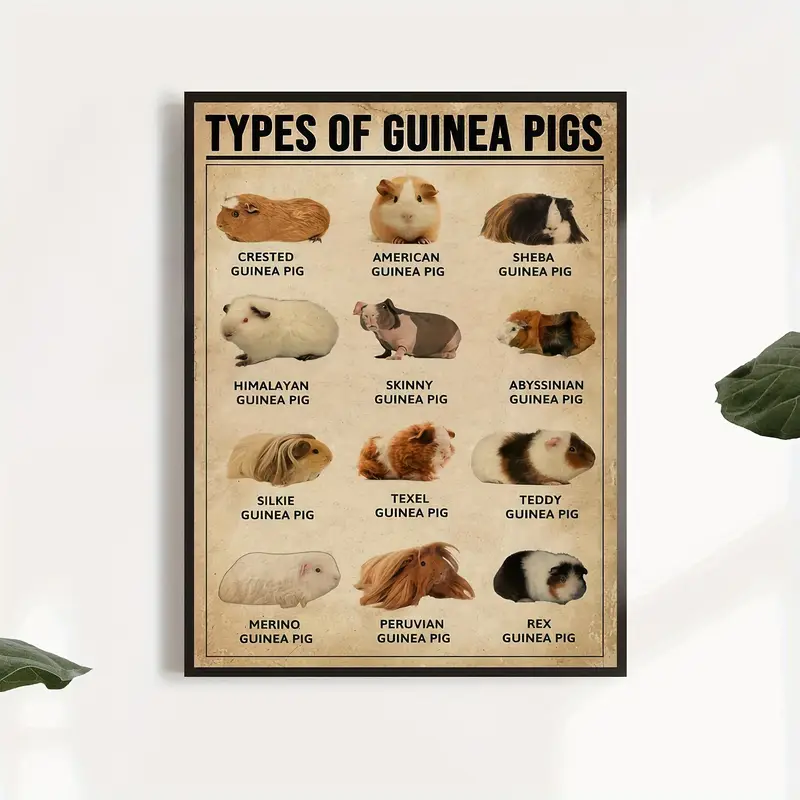This image is a photograph of a vertically framed poster, designed like an infographic, showcasing various types of guinea pigs. The poster is mounted on a white or off-white wall, although the shadow suggests possible digital manipulation. The poster, which has a thick, dark brown border, features a beige background with the title "TYPES OF GUINEA PIGS" at the top in bold, black capital letters, underscored by a dark black line.

The poster is divided into four rows and three columns, each containing a distinct photo of a guinea pig with its name labeled underneath in black capital letters. The top row displays a brown Crested Guinea Pig on the left, a brown and white American Guinea Pig in the center, and a long-haired black, white, and brown Sheba Guinea Pig on the right. The second row includes Himalayan Guinea Pig, Skinny Guinea Pig, and Abyssinian Guinea Pig. The third row shows Silky Guinea Pig, Texel Guinea Pig, and Teddy Guinea Pig, while the fourth row features Merino Guinea Pig, Peruvian Guinea Pig, and Rex Guinea Pig.

The guinea pigs vary in appearance, with colors ranging from white, brown, and black to gray, and hair length from short to long. Notably, one guinea pig is hairless, standing out with an unusual appearance. Additionally, two dark green leaves are visible: one in the bottom left corner and another in the middle right edge, suggesting room decoration or background elements.